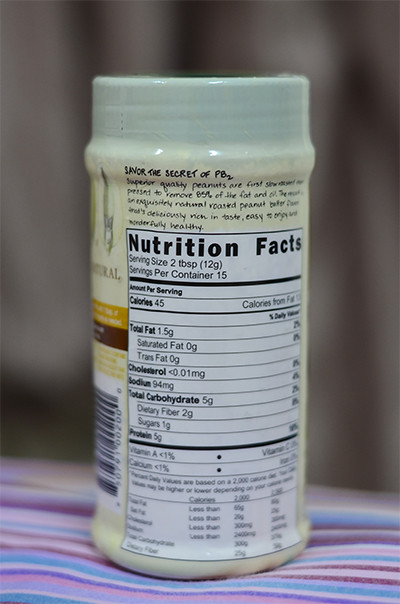This photograph captures the back of a small jar of peanut butter, prominently displaying its nutrition facts within a white rectangular area. The black writing on the label specifies that the serving size is two tablespoons, and the jar contains approximately 15 servings. Below the serving information, detailed nutritional data is provided, including the amounts of total fat, cholesterol, sodium, and other nutrients such as vitamins and minerals.

On the left side of the jar, where it curves, a black and white barcode is visible. The peanut butter label itself is a light yellow color, and the jar is topped with a light green cap. The label appears to be made of plastic, featuring dotted lines indicating where to break the seal to open the jar.

The jar is placed on a cloth with stripes in various shades of pink, purple, blue, and red, adding a colorful backdrop to the scene.